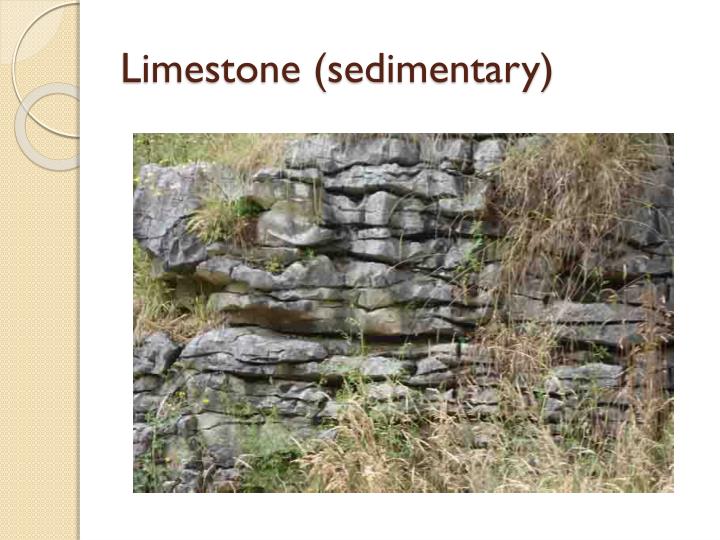This image, depicted in a Microsoft PowerPoint presentation slide with a white background and a burgundy heading that reads "Limestone (Sedimentary)," showcases a well-worn limestone wall in the wild. The slide design includes a tan sidebar with a hollow gray half-circle and additional tan circle graphics. The focal point, however, is the large photo of the weathered limestone wall. 

The wall, composed of several layers of gray sedimentary rock, reveals noticeable horizontal cuts and dark crevices between the layers. This natural structure is partially obscured by various grasses and weeds, some green, some yellow, and some brown, draping over and growing through the rock crevices. The setting appears to be outdoors on a sunny day, with the rock formation situated on a slope or hill, indicative of a natural landscape rather than a maintained garden or park.